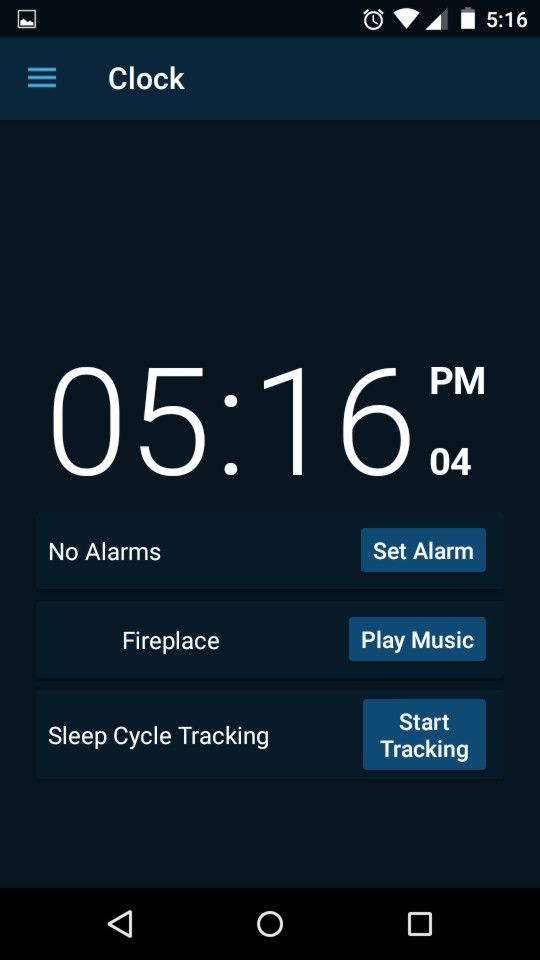Screenshot Description:

The image is a screenshot of a digital interface set against a completely black background. At the top, a blue bar is positioned directly beneath the time display. Written in white text is the word "Cloth," which is accompanied by three horizontal blue lines situated just to its right. Below this header, the screen is primarily dark. Centered prominently in white text is the time "5:16 PM." 

A section below the time indicates "No Alarms," alongside a button that offers the option to "Set an Alarm." Further down, various buttons and options are displayed, including "Fireplace," "Play Music," and "Sleep Cycle Tracking." An interactive option labeled "Start Tracking" is also available.

In the lower portion of the screenshot, there are three distinct icons: a square, a circle, and a triangle, each positioned in a row. These icons likely serve as navigational or functional buttons within the interface.